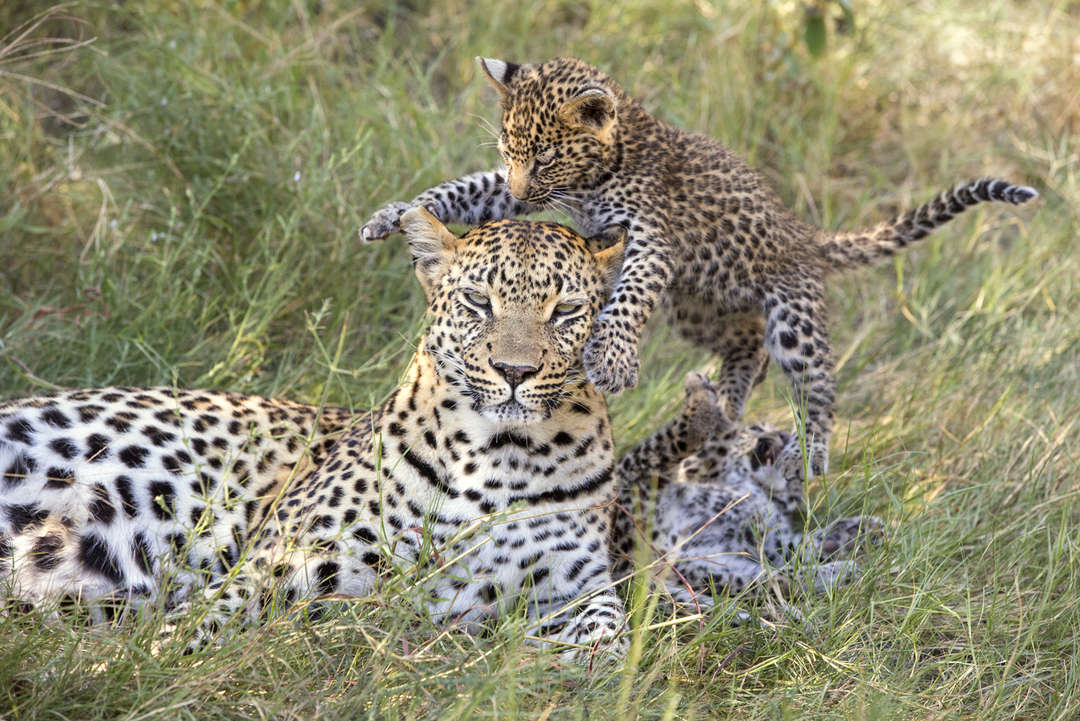In the golden light of what appears to be either sunrise or sunset, a serene meadow with a mix of green and tan grasses forms the backdrop for a captivating scene. A mother leopard, with a striking yellow coat adorned with black spots and a white underbelly, lounges calmly on the grass, her watchful yellow eyes gazing forward. Her tranquil demeanor remains unfazed by the antics of her two playful cubs. One cub, matching its mother's coloring, is captured mid-leap as it pounces from behind, aiming for her head. Meanwhile, the second cub lies on its back in the grass beneath the mother, its small paw raised and mouth open as if caught in the midst of play. The mother's white whiskers and the cubs' lively behavior are sharply detailed, thanks to the fast shutter speed used in capturing this moment. The scene exudes warmth and a sense of familial interaction, enriched by the natural beauty of the glowing landscape.